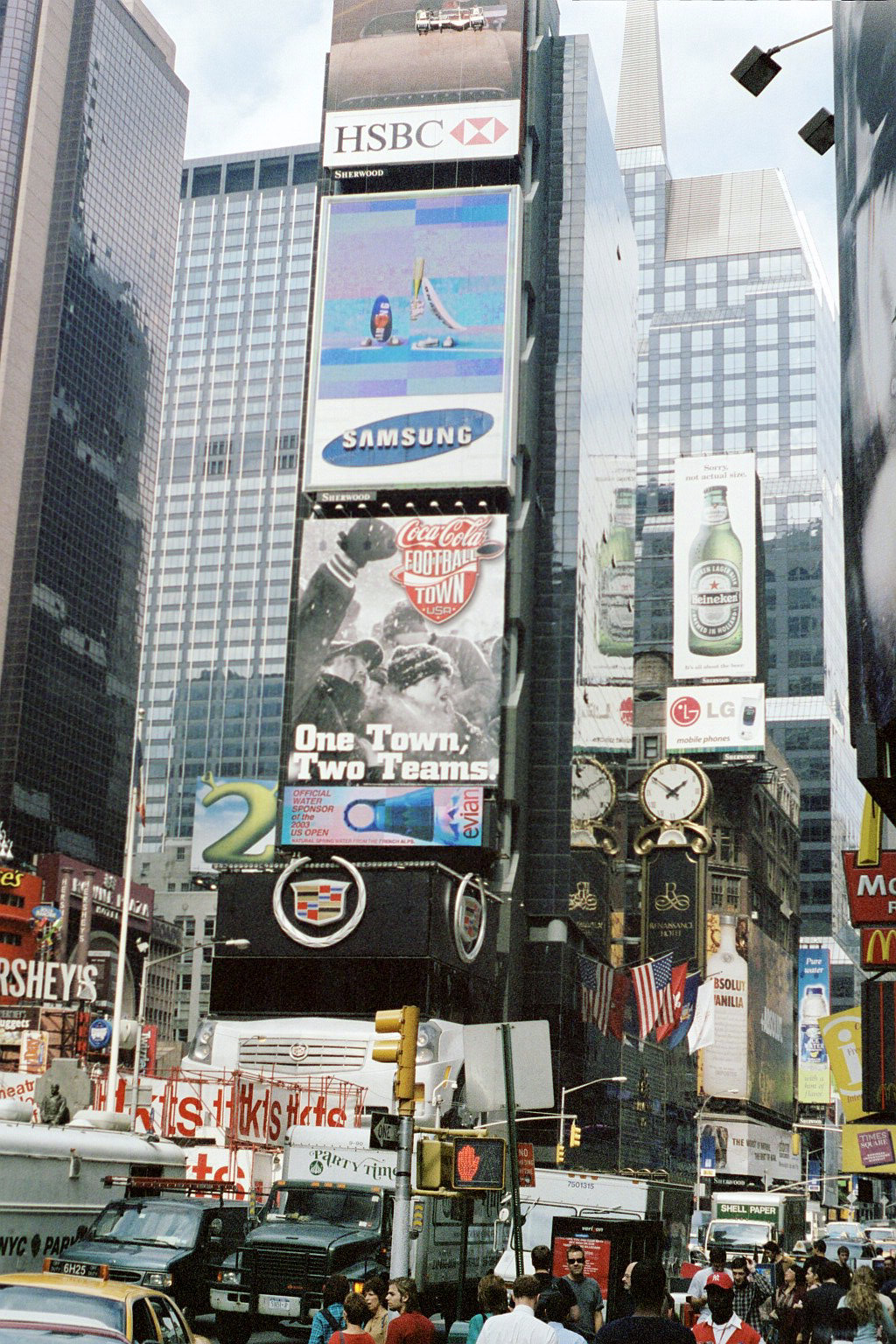The image captures the bustling atmosphere of Times Square in New York City. Dominating the scene is a tall and narrow tower adorned with numerous vibrant billboards: HSBC at the top, Samsung in the middle, and a black-and-white Coca-Cola Football Town advertisement featuring two fist-pumping men with the slogan "One Town, Two Teams". Beneath these, there's an Evian billboard, and the base of the structure sports a Cadillac logo. Scattered around the background, additional advertisements can be seen, including those for Heineken, LG, Hershey’s, Reese's, McDonald's, and Absolut Vodka. The iconic TKTS booth stands at the bottom of the tower, surrounded by dense traffic consisting of taxis, trucks, food vans, and cars moving toward the camera. The streets are filled with pedestrians navigating through the hustle and bustle, set against the backdrop of towering skyscrapers under an overcast sky.